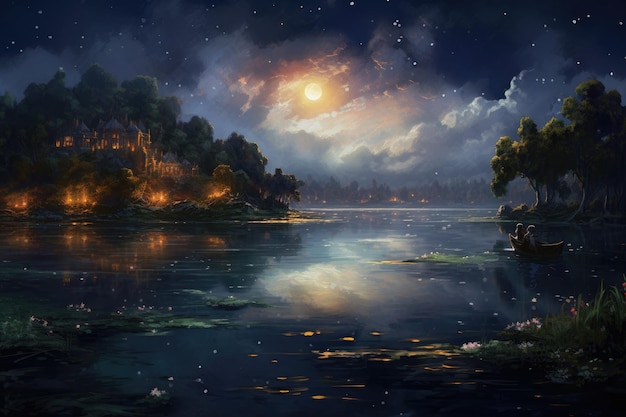This stylized, fantastical landscape appears to have been created by AI, featuring a nightscape of improbable dimensions and vivid colors. Dominated by dark midnight blues, the scene showcases a strikingly bright full moon that shines almost as intensely as the sun, illuminating an expanse of elaborate white clouds and a sky filled with glaring white stars. Below, water reflects the celestial glow, stars, and moonlight, creating a shimmering effect. Flames hover mysteriously on the water's surface, adding an ethereal element.

In the center of the image, a small island houses several structures that seem to be engulfed in flames, suggesting a potential spread down towards the water. A canoe with two people sitting side by side navigates the water, a rare sight in such a craft. Surrounding the scene are trees and bushes casting shadows into the water, contributing to the intricate reflections. The scene also features lily pads, stone-like formations, and possible waterfalls, adding to its fantastical nature. The landscape is enriched with subtle contrasts of white and green hues, glowing lights, and a surreal night sky that captivates with its otherworldly beauty.